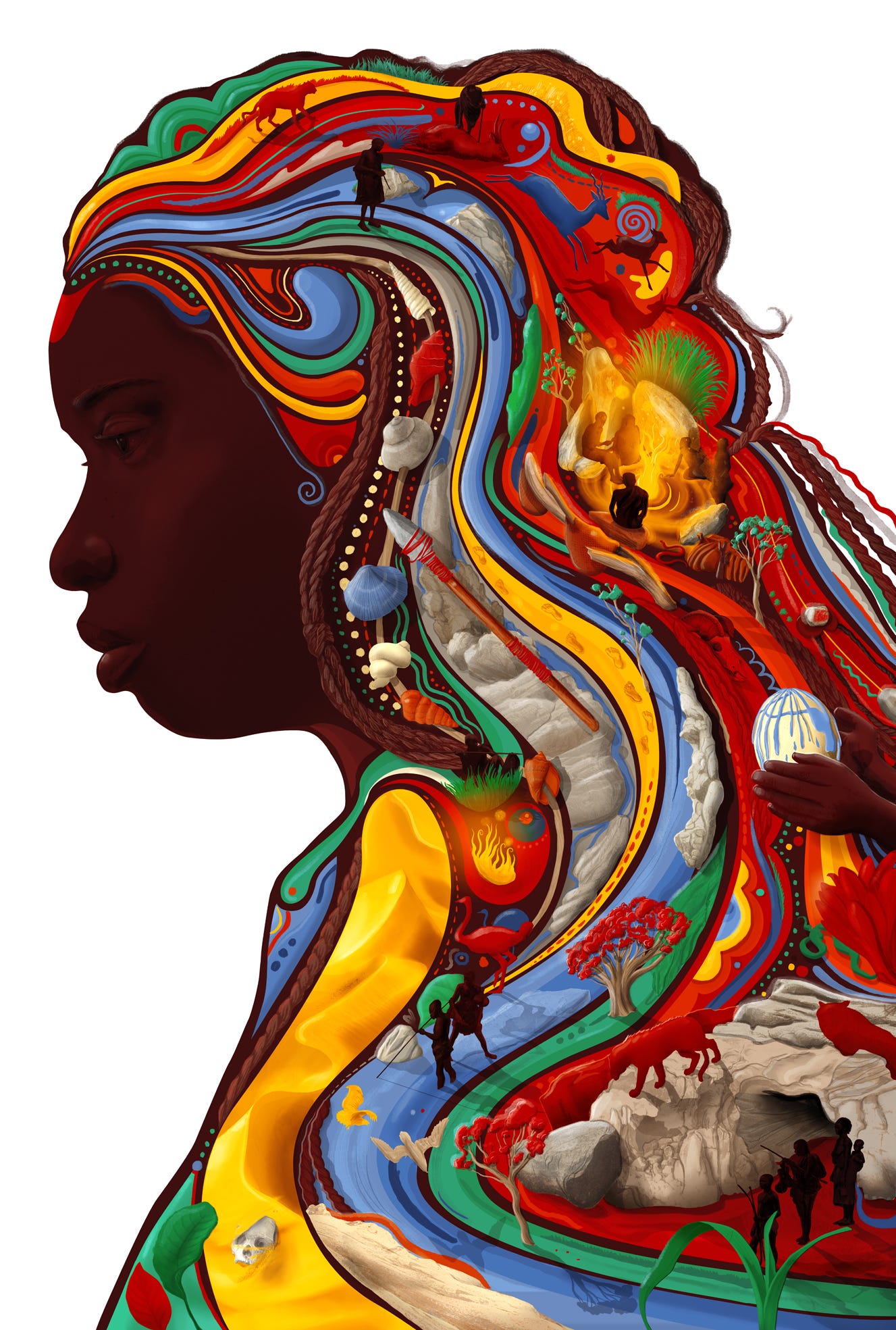This image is a beautifully detailed work of art, showcasing a young African-American woman in profile, her serene expression suggesting deep thought. Her hair is depicted as a cascading array of vibrant colors—blue, green, red, and yellow—filled with intricate imagery. Among the swirling patterns, one can discern silhouettes of people, animals like gazelles and antelopes, and various objects such as seashells, a spear, and a skull. Further detail reveals a tree with bright red foliage, a creek with people standing in it, a wild cat atop a cave, and individuals camping around a fire. A recurrent element throughout the composition is a river interconnecting these images, alongside clouds and green trees. Notably, there's also a hand holding an egg or orb, symbolizing perhaps a cultural or personal significance. The integration of these diverse elements into her hair creates a mesmerizing and colorful portrait that speaks volumes about her identity and heritage.